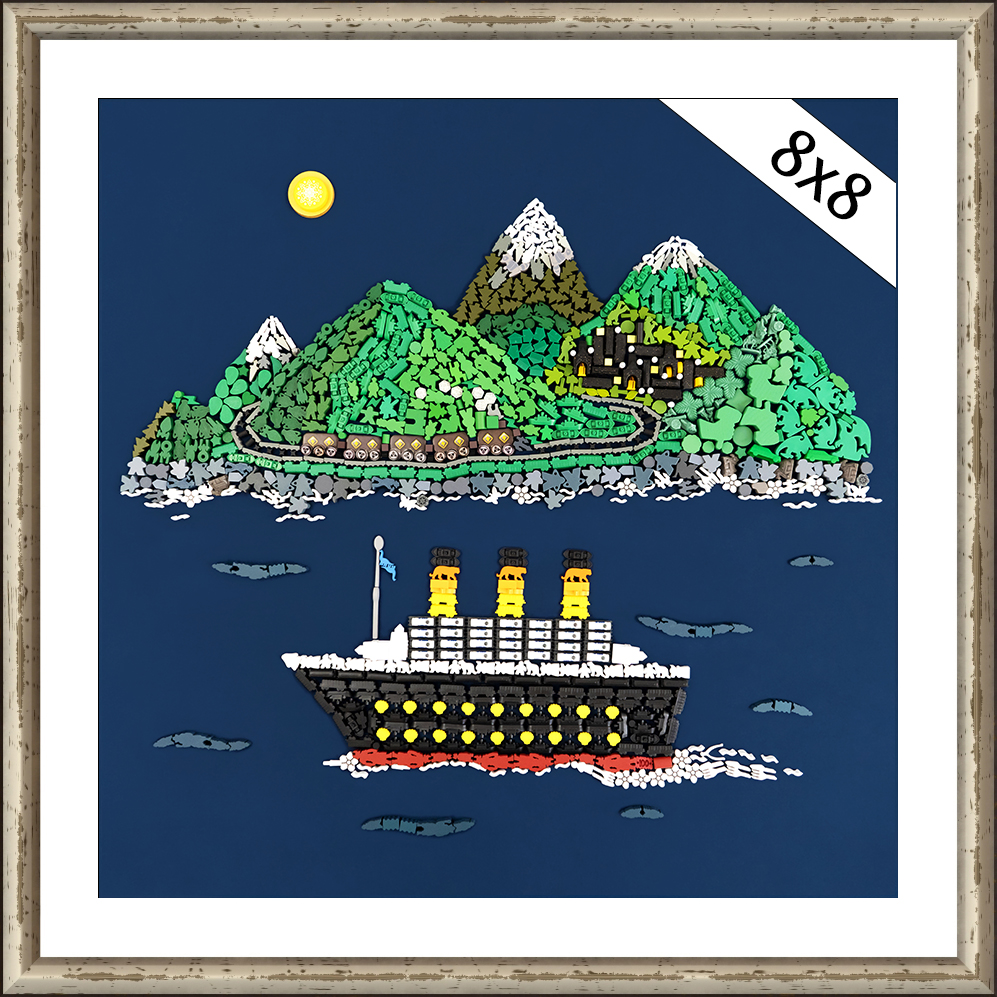This detailed painting, possibly AI-generated or hand-crafted with unique, rotated object shapes like trees and animals, is encased in a square, grey frame and adorned with white borders. Central to the composition is a blue sea with intricate markings depicting water movements. Sailing on the sea is a brown ship, reminiscent of the Titanic, equipped with a blue flag and several yellow and brown tower-like structures. The ship's hull has shell-shaped, yellow holes. Behind the ship, an island emerges with a train track traversing tree-lined mountains. The brown train, comprising five compartments and adorned with yellow blocks, emits white smoke as it progresses along the tracks. Above, a bright yellow sun or moon illuminates the scene from the top left corner, while an 8x8 inscription on a white strip occupies the top right corner, likely indicating the image’s dimensions. The entire image conveys the essence of an imaginative, blocky, computer-generated visual experience, blending maritime and mountainous elements into a cohesive, vibrant work of art.